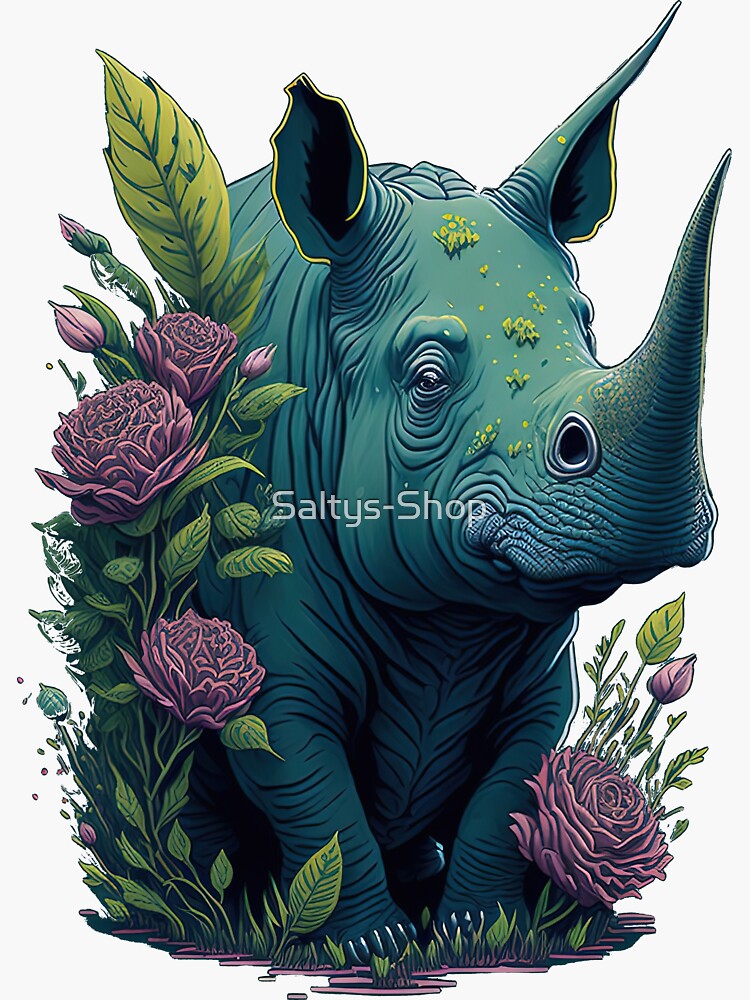The image is a vibrant piece of digital art featuring a bluish-green rhinoceros, partially obscured by lush foliage adorned with pinkish-purple wildflowers. The rhino, detailed with definition lines and speckled with what appears to be pollen or moss on its head, is depicted walking towards the viewer with its head tilted slightly to the right. This positioning showcases the left side of its face and the prominent single horn on its nose. The ears of the rhinoceros are notably outlined in yellow and are standing upright, adding a touch of whimsy to its appearance. The scene has a fantastical quality, with the rhino appearing inquisitive yet benign as it peers through the greenery. The foreground and left side of the image are rich with green leaves and vibrant flowers, creating a jungle-like atmosphere. Overlaid in the center of the graphic is white text that reads "Salty's Shop," indicating that the image might serve as an advertisement or representation of this locale. The detailed and colorful portrayal of the rhino and its surroundings creates an engaging and immersive visual experience.